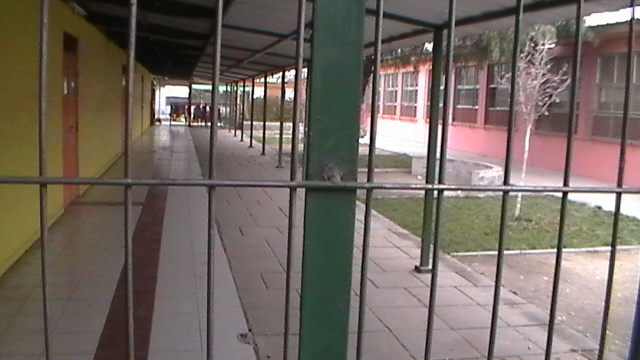The photograph captures a view from outside a gate characterized by vertical and horizontal silver bars, with a prominent green metal girder centrally visible. Through the gate, a meticulously detailed scene unfolds within what appears to be a courtyard of a school or perhaps another institutional setting. Immediately inside, a light gray brick sidewalk stretches forward, flanked on the left by a white-tiled walking area adorned with a maroon stripe. This tiled path runs adjacent to a prominent yellow wall, punctuated by several orange doors, suggesting entrances to rooms or facilities. Towards the end of this brick sidewalk, some distant figures can be faintly discerned, adding depth to the scene. On the right side of the courtyard, there are several small, square green plots housing bare trees, contrasting with the surrounding architecture. Further right, a pinkish-red building wall featuring numerous windows leads the eye upward, complementing the color complexity of the scenery. The overall composition is a blend of vibrant architecture and organized pathways, evoking a sense of order and purpose.